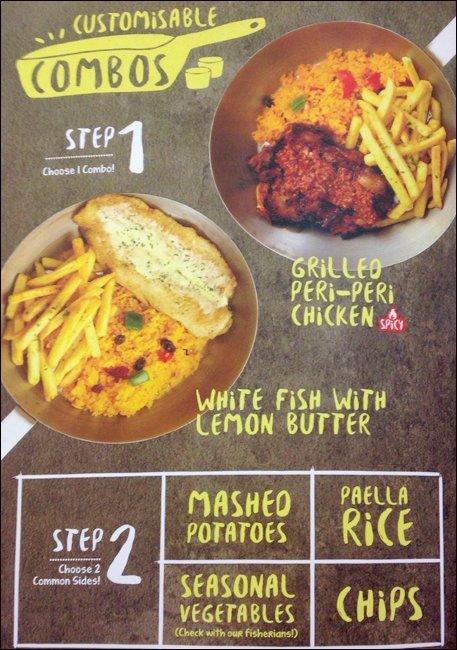The image is a vertical rectangular menu page with a granite-colored dark gray or black background. At the very top, there's a stylized cartoon frying pan on its side with the word "Combos" inside it. Above the pan, yellow text reads "Customizable," and below it in white text it states "Step 1: Choose 1 Combo."

The menu showcases two dishes in skillets positioned diagonally from each other, centered toward the top. The top right skillet contains fried rice, french fries, and a grilled peri-peri chicken breast, labeled in yellow text as "Grilled Peri-Peri Chicken," which is noted to be spicy. The bottom skillet has fried rice, french fries, and a slice of white fish with lemon butter, labeled "White Fish with Lemon Butter."

Below the skillet dishes, additional menu instructions detail "Step 2: Choose Your Sides," which include options for mashed potatoes, seasonal vegetables, paella rice, and chips (french fries). The color palette of the menu includes yellow, red, green, black, brown, beige, silver, gray, and white, creating a vibrant and appetizing display.